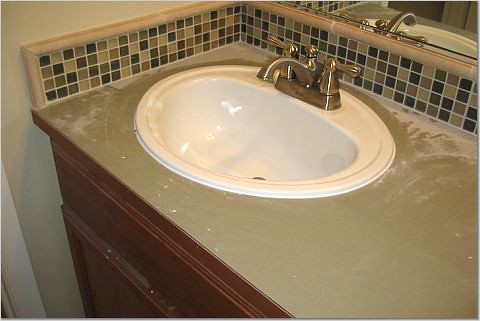A dusty, dated bathroom vanity occupies a small portion of the image, hinting at recent renovation activities. The vanity features a dark tan Corian countertop, partially obscured by a layer of dust, suggesting sanding work. Embedded in the countertop is an oval, white porcelain sink equipped with a brushed silver-tone faucet with dual handles. Above the counter, an abstract mosaic of small black, tan, and brown tiles is arranged with white grout and framed with wooden trim. The backdrop includes tan walls and white woodwork visible on the left side. The dark brown woodwork of the cabinet underneath the sink adds a stark contrast to the light-colored dust that blankets the surface. Evidently, an attempt was made to clean; a single swipe reveals a clearer, circular patch amidst the dust-coated counter, indicating an ongoing effort to restore cleanliness.